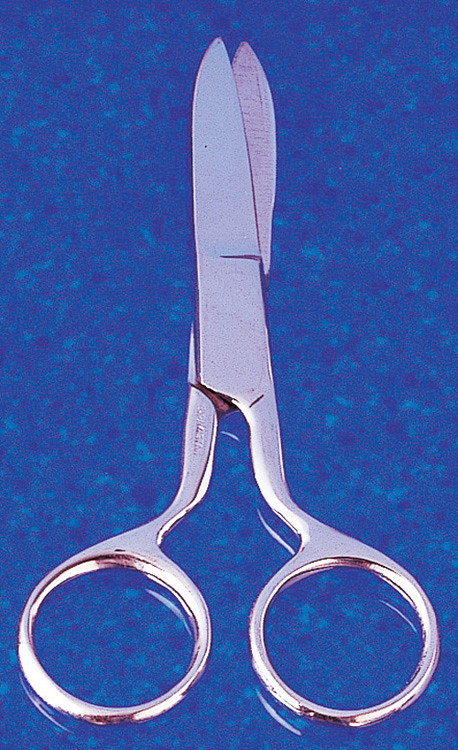In the image, a pristine pair of stainless steel scissors lies on a blue background, which appears to be a soft, textured surface possibly resembling felt, carpet, or even water with varying shades of blue and subtle lines. The silver metal scissors stretch from the bottom, where their round, circular handles are located, to the top, where the blades are slightly ajar. The image is closely zoomed in, providing a clear view of the scissors' clean, rust-free appearance. The blades are both thick and thin, suggesting they might be specialized for tasks like cutting hair or performing delicate procedures.